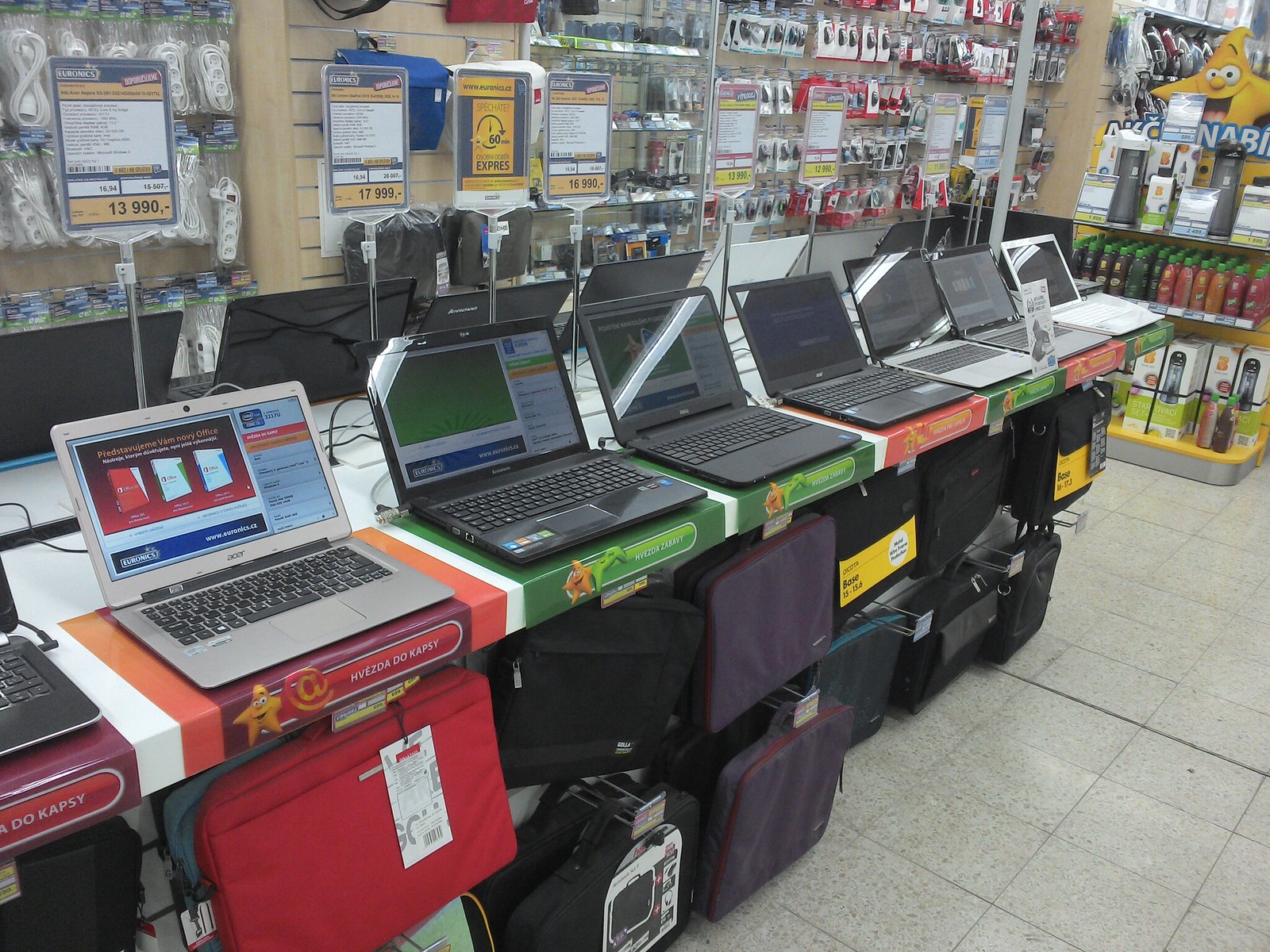The image captures the interior of an electronic store, bustling with various electronic gadgets and accessories. The focal point includes a display of multiple laptops, predominantly silver, black, and one white, each sitting on individual white stands with red tiles underneath. Below the laptops, there are laptop bags for sale in shades of red, white, and black, neatly hanging on racks. The backdrop, a light brown wooden wall, is lined with a plethora of electronic parts, including cables, chargers, and other accessories, all in plastic packaging. On the right side, the scene reveals blue and white bags, as well as a variety of bottled drinks and an enigmatic device on the far end. The gray tile floor adds a contemporary touch. Sprinkled around the store are price tags featuring both dollar amounts and a foreign currency. Dominating the visual field is a recurring yellow star-shaped mascot, accompanied by visible signage with phrases like "HV-EZDA DO KAPSY" and the word "express." The laptops, open and displaying varied content on their screens, stand as the centerpiece of the store's offerings, completing this vibrant snapshot of a modern electronics retailer.